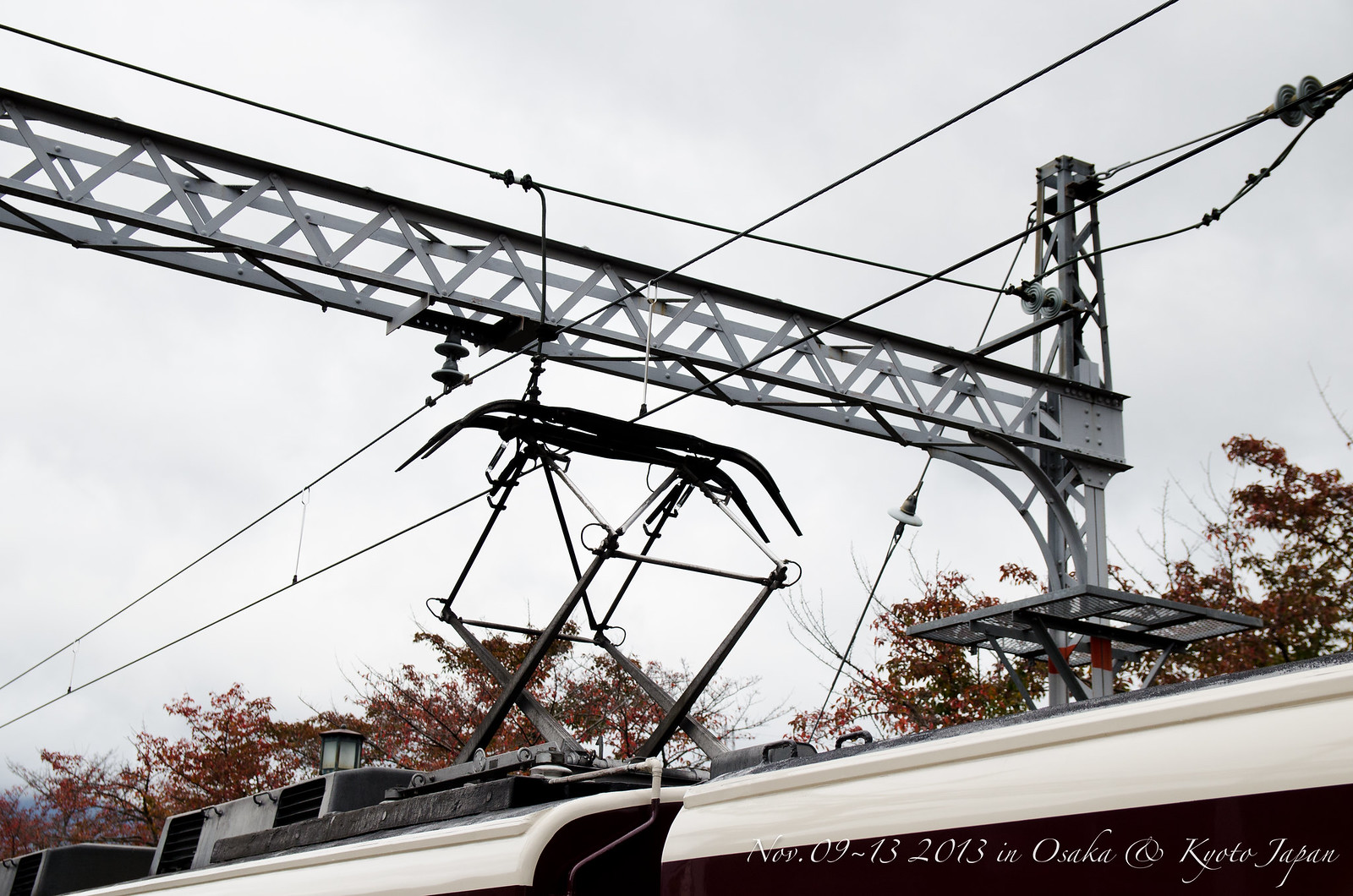The image captures an outdoor scene featuring the top of a maroon-bodied tram with a white roof, connected to various metal beams and thick cables. This intricate setup includes pulleys and a steel support frame reminiscent of heavy machinery for lifting objects. The cables run both vertically and horizontally, indicating functionality as part of the tram's movement or support system. The background displays a cloudy, white sky and autumnal trees with orange and red leaves, suggesting a late fall setting. In the bottom right corner, white lettering reads "NOV.09-13 2013 in Osaka, Kyoto, Japan."